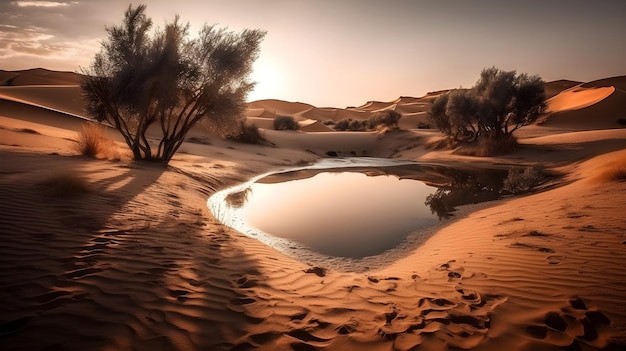This AI-enhanced image captures a serene desert oasis featuring a small, tranquil pond or pool of water nestled among rust-colored, terracotta sand dunes. The calm, black surface of the pond reflects the sparse, brown trees encircling it, adding a mysterious depth to the scene. In the background, undulating sandy hills stretch across the horizon. The sky above is a muted gray, adorned with a mix of white clouds clustered towards the left side. This evocative desert landscape juxtaposes the stark, barren beauty of the dunes against the tranquil stillness of the black pond.